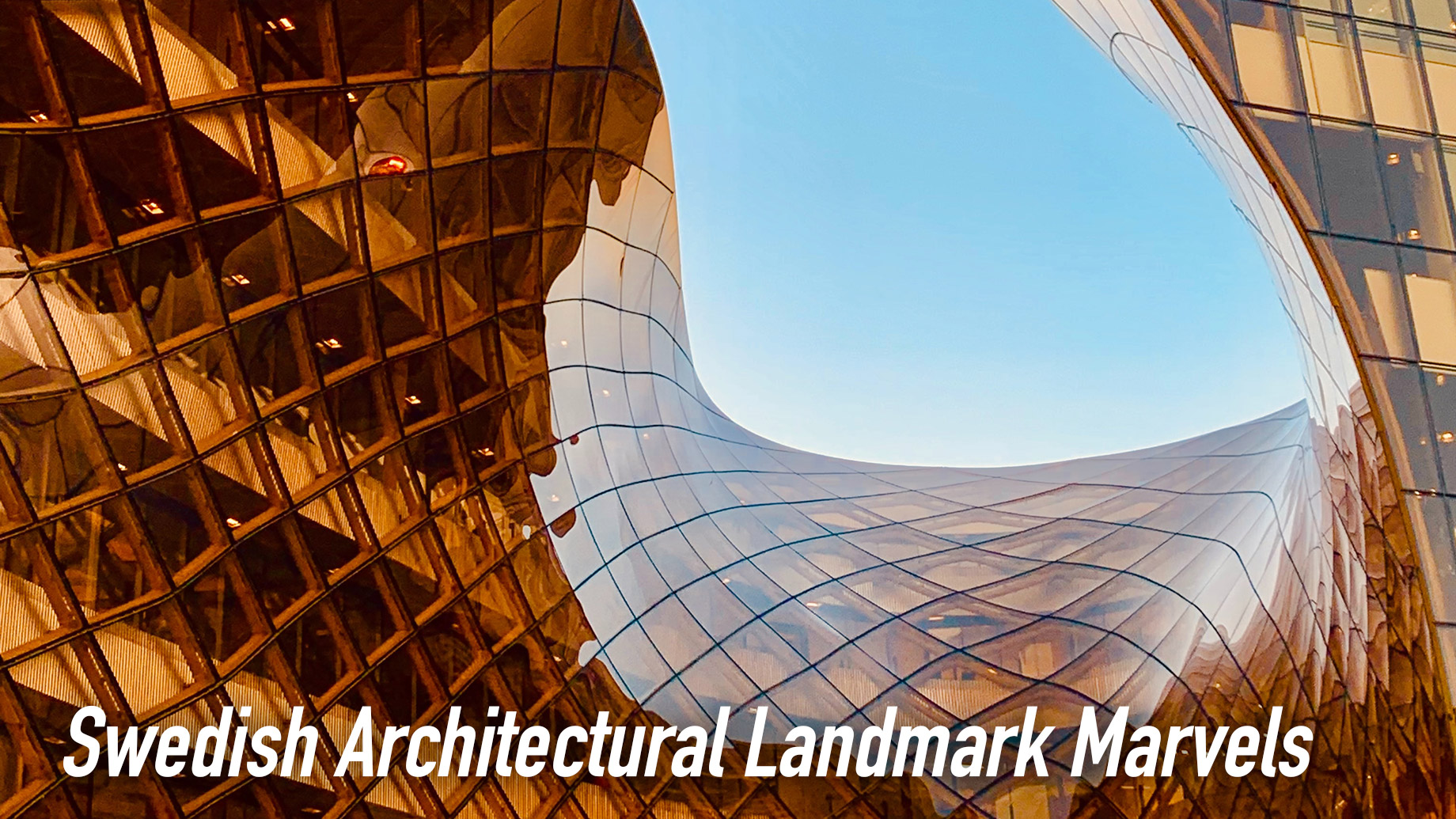The image is a color photograph, taken in landscape orientation, of the exterior of a large building that features an innovative and captivating design. The building is constructed with a wooden framework forming a honeycomb-like texture, and it is covered in amber-colored, reflective glass panels. The structure warps in a smooth, wavy manner, wrapping around from the top left, across the center, and back up to the top right in a U-shape, creating a surreal, abstract pattern. From the ground-level perspective looking up, there's a small circle of blue sky visible in the upper center of the image. This sky patch emphasizes the building's unusual, encapsulating architecture. A flat section of glass in the upper right corner faces the viewer, contrasting with the warped shape of the rest of the structure. Across the bottom of the photograph, in bold white letters, it reads "Swedish Architectural Landmark Marvels," highlighting the unique and impressive nature of this modern architectural feat.